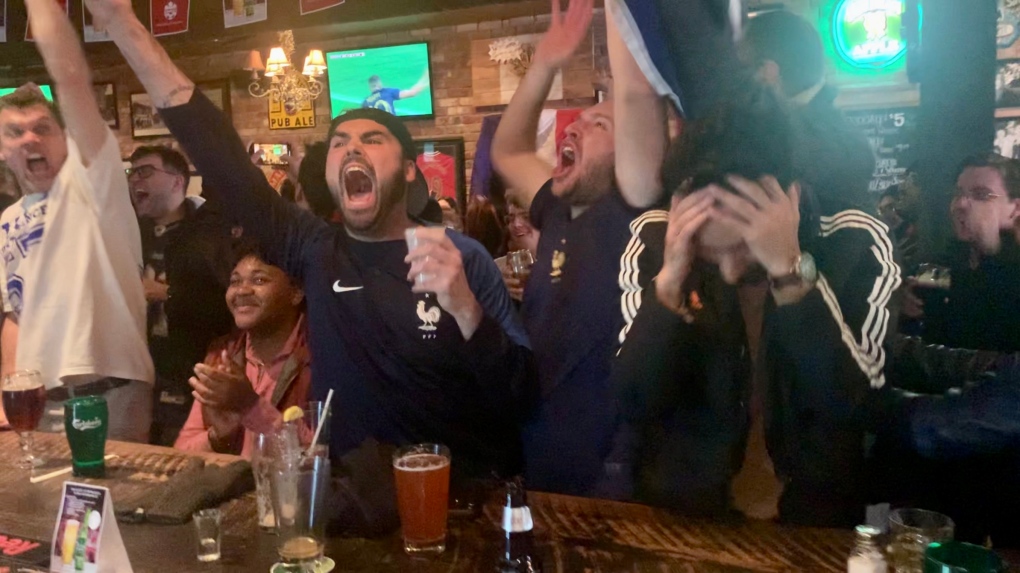In this vibrant, full-color indoor photograph, likely taken by a bartender behind the bar counter, a group of exuberant men are captured amidst a jubilant celebration. The atmosphere is illuminated by artificial light, emphasizing the lively and colorful setting of the bar. Dominating the left side of the image, most of the patrons are standing with their arms raised, their mouths open in ecstatic cheers, reacting to an exciting moment in a soccer match displayed on a television screen near the top left. Among the cheering crowd, one man in the center left is seated, clapping his hands, while another man on the center right, dressed in a black Adidas jacket with white stripes, sits despondently with his head in his hands, wearing a watch on his left wrist. The scene is accented with various bar items scattered along the bottom of the frame, including salt shakers, a beer bottle, a nearly full glass of beer, a clear glass with straws, a green glass, and a shot glass. A neon sign glows in the upper right corner, adding to the vibrant energy of this celebratory yet contrasting scene.